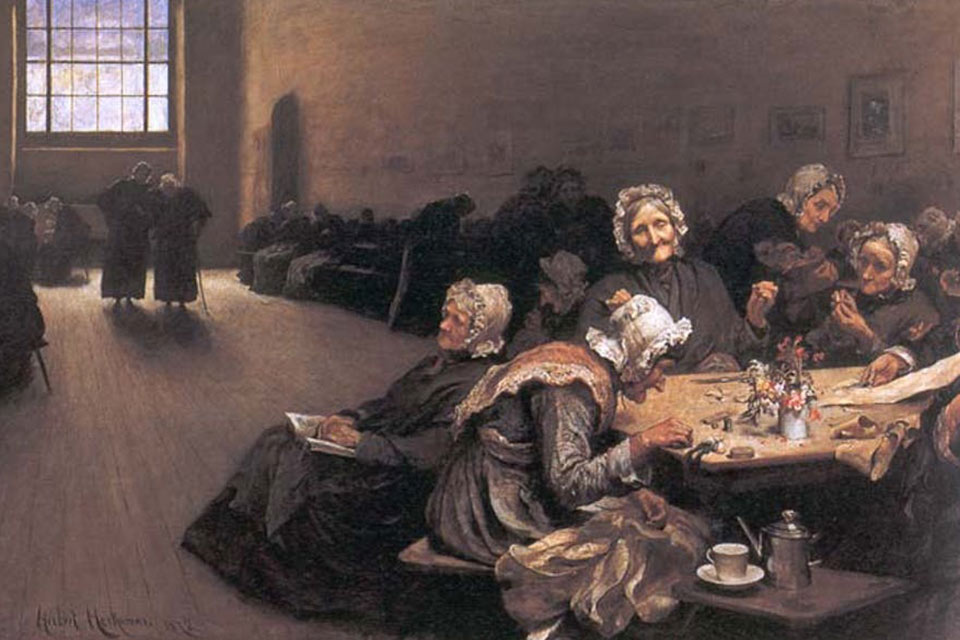This rectangular image, resembling a painting or a detailed drawing, depicts a scene titled "Eventide" in the Westminster Union by Hubert von Herkimer. The image appears as a paper print, wider than it is tall, and showcases a group of elderly women dressed in gray or black long dresses with white bonnets. They gather predominantly around a table adorned with a teapot, a teacup, and some wilted flowers. In the foreground, one woman reads a book, reclined in her chair as though she is sleeping, while another picks up crumbs from the table. One woman, possibly sewing or performing a small task with her hands, adds to the quiet, domestic atmosphere.

The background, which is a grayish beige color, features additional groups of women, some seated at tables or on a couch, contributing to a sense of community yet solitude. The lighting is dim, with none of the women particularly in focus except for the main group near the right side of the image. Further enhancing the serene and aged ambiance is a large picture window in the back left-hand corner and faint images of portraits lining the wall from the window to the right side. Among the background figures, one woman holds a cane as she walks, accompanied by another who seems to be assisting her. This deeply detailed scene evokes a sense of tranquility and bygone eras, reminiscent of 17th or 18th-century servant gatherings.